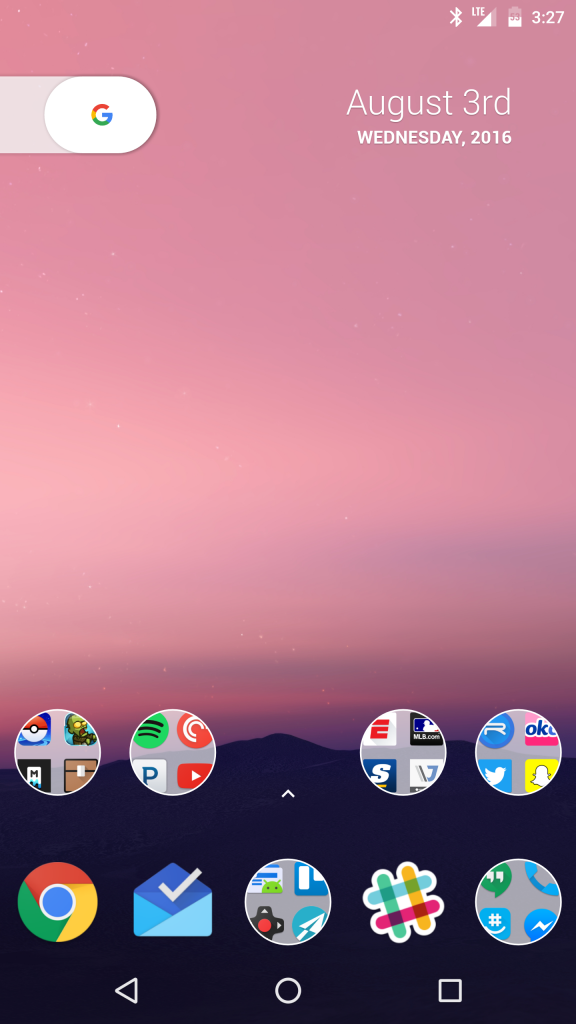A screen capture of a smartphone display showcases a visually stunning sunset with a sky bathed in gradients of salmon and pink, occupying the top two-thirds of the image. In the upper right corner, status icons are visible, including a Bluetooth symbol, an LTE signal triangle with three bars, and a battery indicator at 53%, while the time is displayed as 3:27 PM. Below that, in larger, bold white letters, the date reads August 3rd, Wednesday, 2016. On the left side, a Google slide-in oval button with a white background featuring the multicolored 'G' logo is seen. The bottom section of the screen displays various app icons. The top row consists of four folder icons, each represented by a circular white outline. The bottom row includes five icons: the Google app, a blue envelope with a white checkmark, a centered folder icon outlined in white, a colorful Tic-Tac-Toe logo, and another circular folder icon outlined in white on the far right. The bottom third of the image is accentuated by the silhouette of a mountain range, creating a stark contrast against the vibrant, pastel-hued sunset.